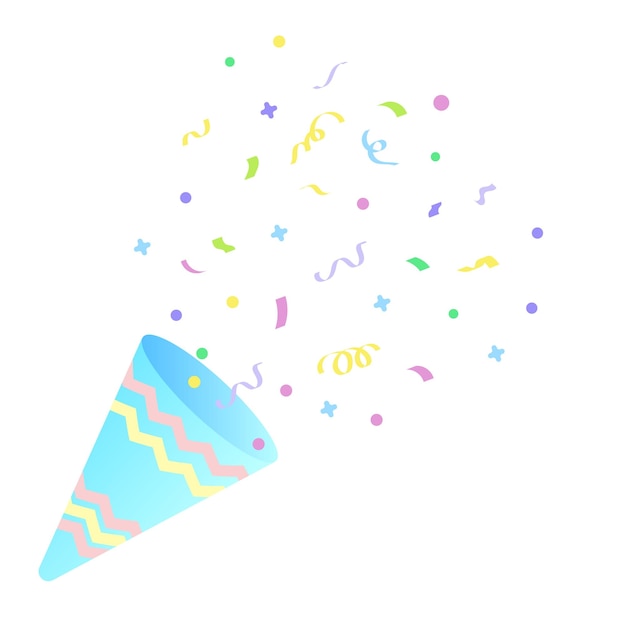This image features a festive, computer-printed party horn on a pure white background. Positioned in the lower left corner, the horn is predominantly blue with zigzag lines in pink, yellow, and orange, wrapping around its body. The top of the horn showcases alternating pink and yellow bands. Bursting from the open end of the horn are various celebratory elements: pink dots, blue Xs, yellow, purple, and blue coils, as well as green semi-circles. These colorful confetti pieces and ribbons float up towards the upper right-hand side of the image, creating a joyous and party-like atmosphere that evokes feelings of happiness and celebration.